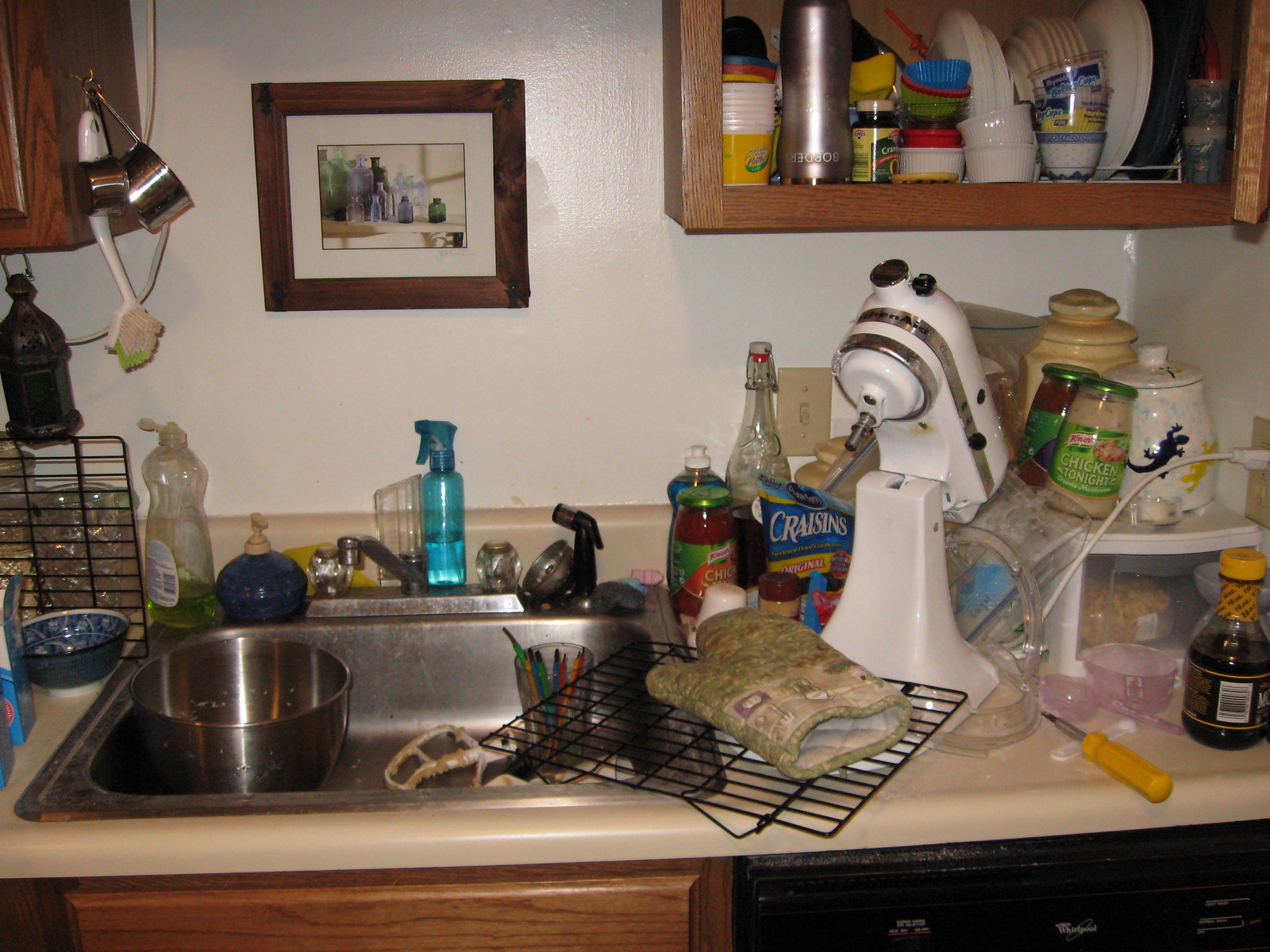A vividly cluttered kitchen is captured in this image, with the sink taking center stage. The sink is filled with various items, prominently featuring a silver mixing bowl positioned on top. Nearby, there are spray bottles and a bottle of dish detergent. The sink also has a black retractable handle, designed to function as a spray nozzle. Perched catty-corner on the sink is a baking rack, adorned with an oven mitt.

To the left of the sink, the clutter continues. A small bowl and a scrub brush hang within easy reach. Above the sink, a brown picture frame with white matting hangs on the wall, though its contents are indiscernible. The right side of the sink area is equally hectic, showcasing the baking rack with the oven mitt once more, accompanied by a large, white mixer. Above this, a shelf is laden with small canisters, contributing to the sense of overcrowding. A yellow knife sits on the countertop among an assortment of items including a jar of spaghetti sauce and a bag of craisins.

Above the counter, a shelf crowded with various dishes comes into view. This shelf holds little bowls, a plate, a silver thermos, and yellow cups, further adding to the overwhelming sense of disarray in this very cluttered kitchen.